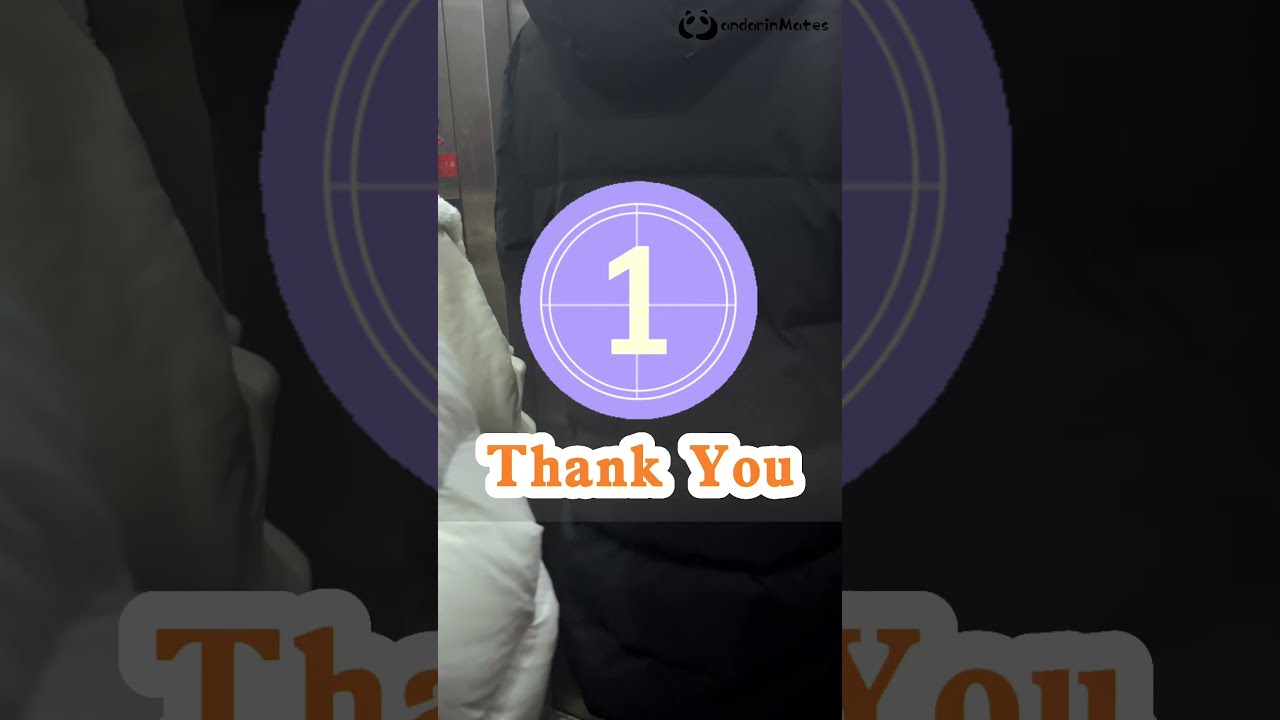The image is a wide, rectangular composition primarily showcasing a tall, central screenshot or photograph flanked by two wider, darker close-up sections of the same image on either side. Central to the composition is the backside of a person wearing a dark gray to black long coat. Adjacent to this person, on the left side, is the edge of a white coat. At the top left of the image, a metal corner is visible. Dominating the middle of the image is a light lavender circle with a bullseye design and the number one inside it. Below this circle, in bold orange font and surrounded by white, is the text "thank you". The backdrop of the image and the close-up side sections are shaded in dark tones, enhancing the visibility and contrast of the central elements. While the setup suggests a PowerPoint or video presentation, the style hints at a countdown setting, perhaps similar to a New Year's Eve ball drop, although this is not explicitly clear.